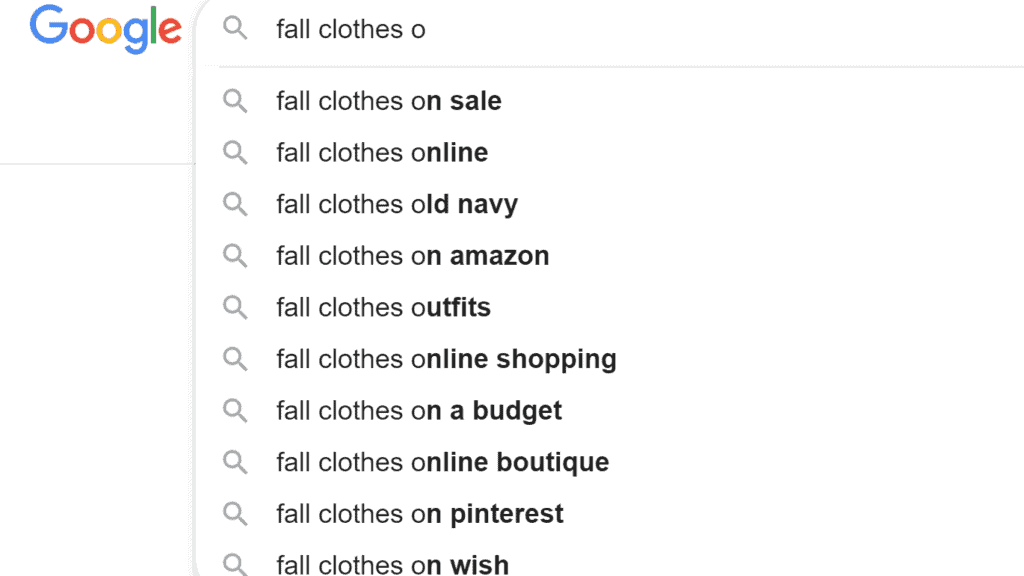The image is a screenshot of a Google search interface. At the top left, the recognizable Google logo is prominently displayed, with the search bar positioned to its right. The user has started typing "Fall Clothes, O" into the search bar. Below the search bar, Google's autocomplete feature provides a list of popular suggested searches related to the entered query. The suggestions, all in black text against a white background, include:

1. Fall Clothes On Sale
2. Fall Clothes Online
3. Fall Clothes Old Navy
4. Fall Clothes On Amazon
5. Fall Clothes Outfits
6. Fall Clothes Online Shopping
7. Fall Clothes On A Budget
8. Fall Clothes Online Boutique
9. Fall Clothes On Pinterest
10. Fall Clothes On Wish

These suggestions indicate trending search terms and common queries associated with "Fall Clothes" as the user begins typing the letter "O."